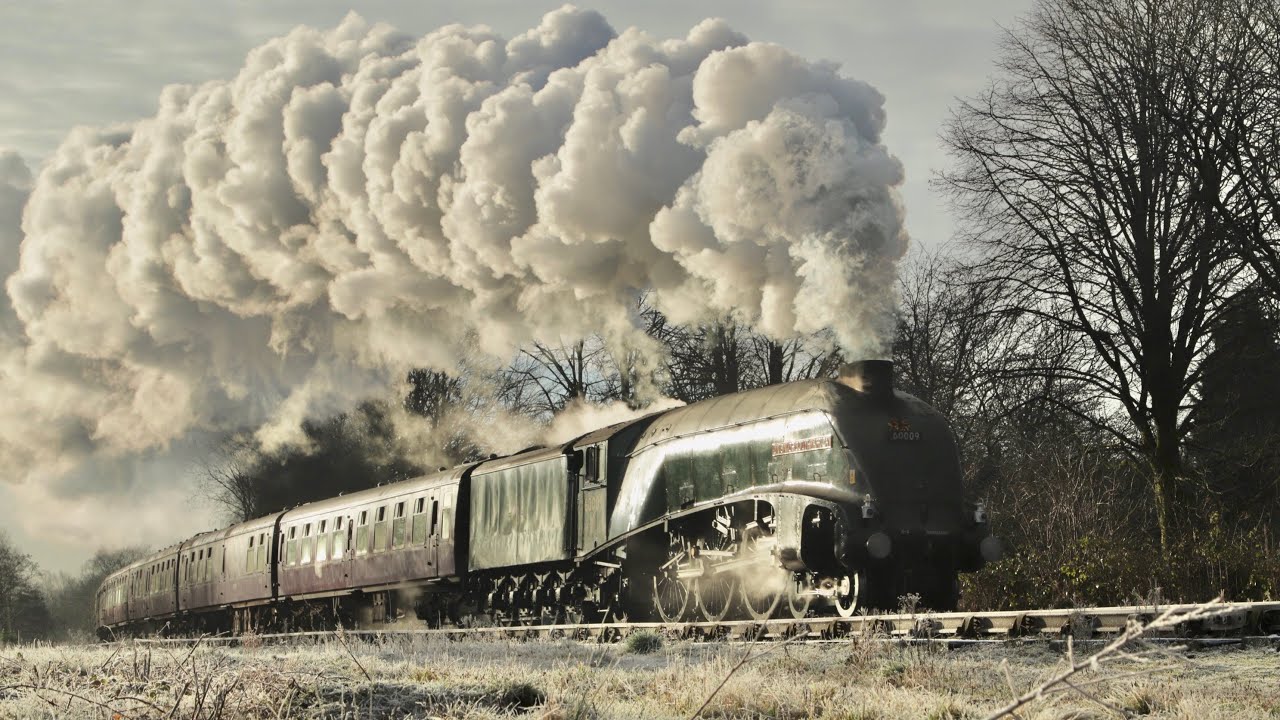In this photograph, we see an old-fashioned, green locomotive with a dome-shaped design, shining in the sunlight as it moves along a track in a rural area. The train is pulling three or more cars, which can be seen curving to the left around a small bend. Great plumes of smoke emanate from the front stack of the engine, trailing back to where it originated. The foreground features grass and branches leading up to the train tracks, while the background has trees that are bare of leaves, suggesting a late fall or winter setting. The overall color palette is fairly monochromatic and drab, with a faded quality that may indicate the photo's age.